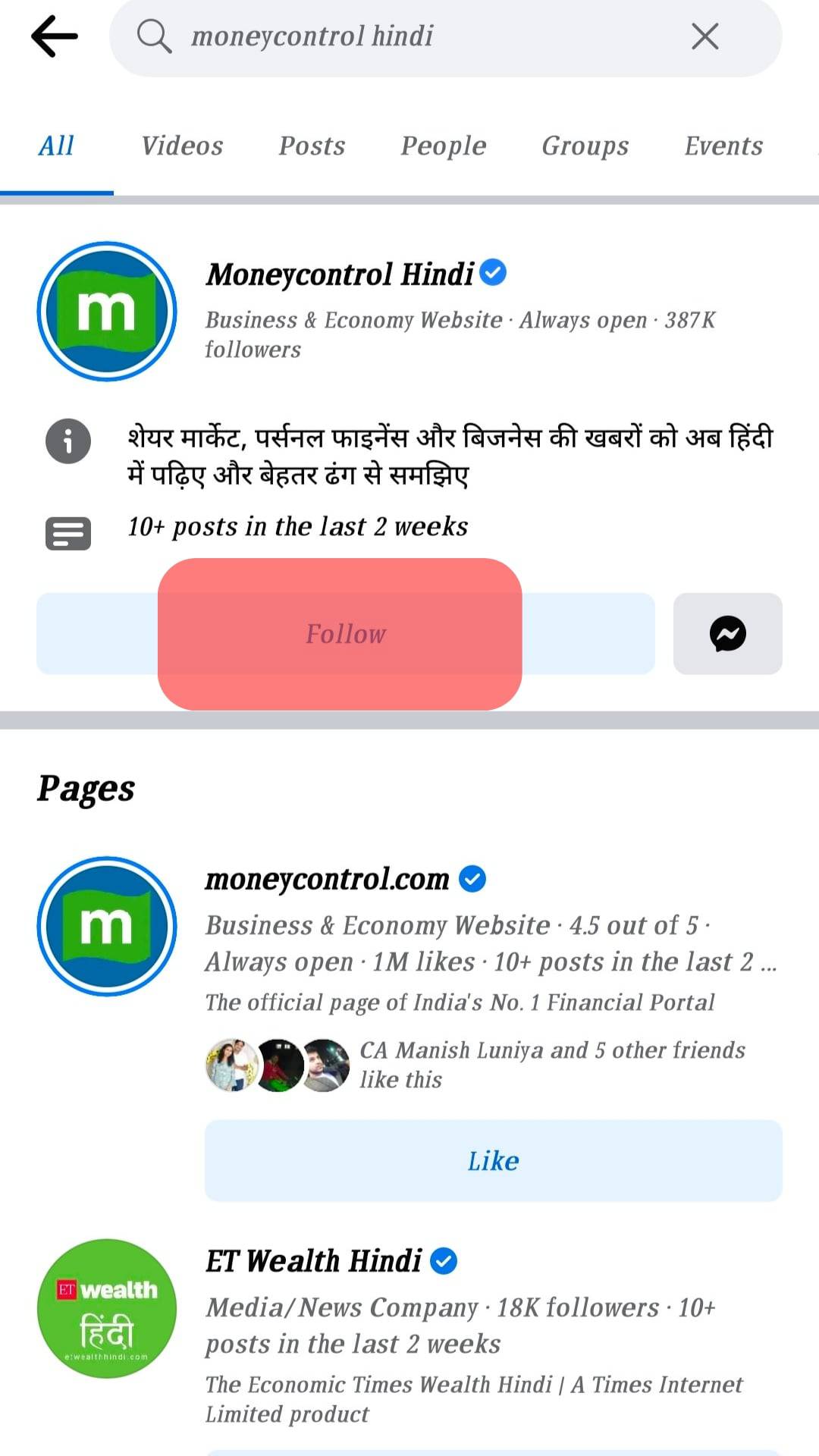This is a detailed screenshot of a website interface with a predominantly white background at the top. At the center of this white section, there is a lightly gray search field with the placeholder text "money control Hindi" written in a gray font. To the left inside the search field, a small magnifying glass icon is visible, while an 'X' icon is positioned to the right.

Directly below the search field, there is a horizontal menu bar featuring several selectable categories. The highlighted selection is "All," but other options include "Videos," "Posts," "People," "Groups," and "Events." Underneath this menu bar, a thin gray line separates these navigation options from the content below.

The first entry below this separator is for "Money Control Hindi," marked with a verified badge. This entry is identified as a business and economy website and is noted as always open with 387K followers. Beneath this, there are two lines of Hindi script, followed by the text "10+ posts in the last two weeks." Adjacent to this text, to the right side, is a red rectangular button labeled "Follow." Another thin gray line appears below this entry.

The subsequent entry is for "moneycontrol.com," also noted with a verified badge. Similar to the first entry, it is described as a business and economy website, rated 4.5 out of 5 stars, and noted as always open. This entry has 1 million likes.